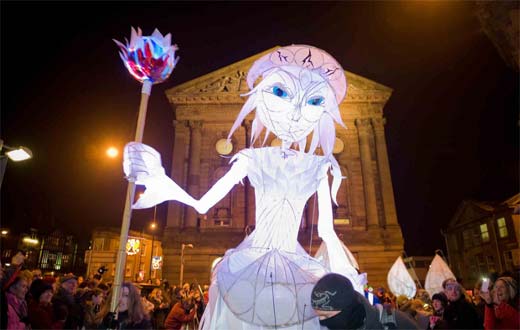In this detailed image, we see an event with a crowd gathered around a striking white structure resembling a Disney princess or perhaps a cartoon villainess. The sculpture stands prominently in the center, holding a staff with a blue orb that has red accents. The figure, with compelling blue eyes and a white dress, wears a crown, adding to its regal yet eerie appearance. A woman appears to be holding the base of the staff. To the right, individuals are seen holding what seem to be leaves or wing-like parts. The backdrop reveals a grand building with large columns, reminiscent of a Tartarian Roman Coliseum, suggesting an ancient, imposing setting. Streetlights illuminate the left side of the image, adding a sense of night-time ambiance. The scene conveys both a mystical and somewhat ominous atmosphere, as the crowd’s dynamic hints at a possible impending action or ritual.